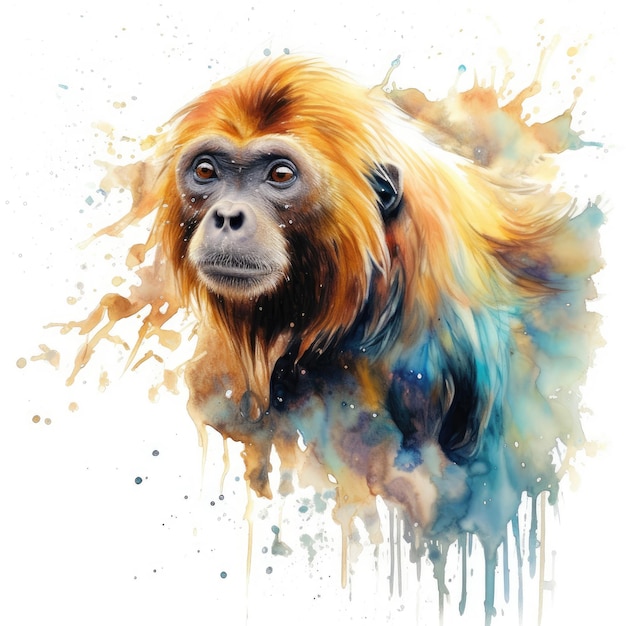This digital artwork features an intricately detailed monkey's face and head, framed against a clean white background. The monkey's fur is a striking mix of reddish, yellow, and orangish-brown tones, giving the impression of a fiery mane. Its expressive brown eyes convey alertness, and a hint of a beard adds texture to its facial features. Adding to the realism, each whisker on its face is meticulously rendered. One black ear peeks out from its vivid hair. Surrounding the monkey, a cascade of watercolor splashes in blues, purples, oranges, and teals blend and drip down the digital canvas, creating an impression of the image dissolving into vibrant colors. The monkey's body subtly fades into a dark teal, blending seamlessly with the artistic background, creating a captivating juxtaposition of detailed digital illustration and fluid watercolor effects.